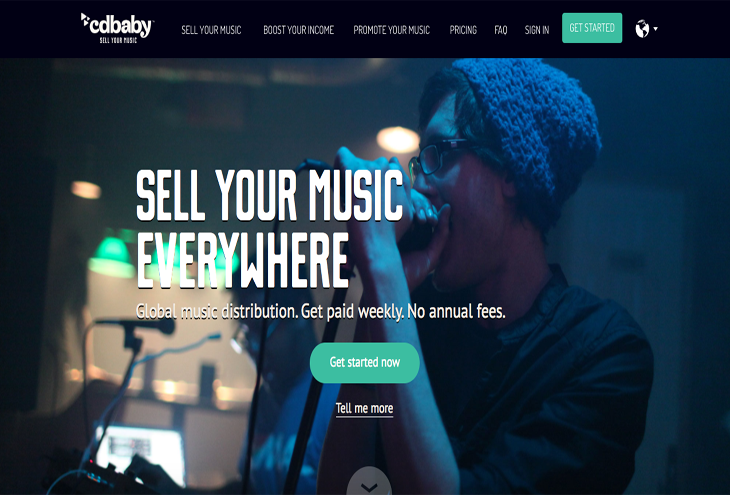A screenshot from the CD Baby website features the prominently displayed slogan: "Sell your music everywhere. Global music distribution. Get paid weekly. No annual fees. Get started now." Below this slogan is a green box with the call to action, "Get Started Now," accompanied by a smaller "Tell Me More" link that likely leads to the terms and conditions.

In the background, a young man appears to be joyfully singing into a microphone. He is wearing a cheerful blue beanie cap, black-framed glasses, and a black shirt. He is surrounded by fellow musicians, contributing to an energetic and collaborative atmosphere. One musician in the far background is playing the guitar, while another individual with a microphone stands next to him, seemingly focused on either a keyboard or another user interface. The scene captures the vibrant and inclusive essence of music creation promoted by CD Baby.